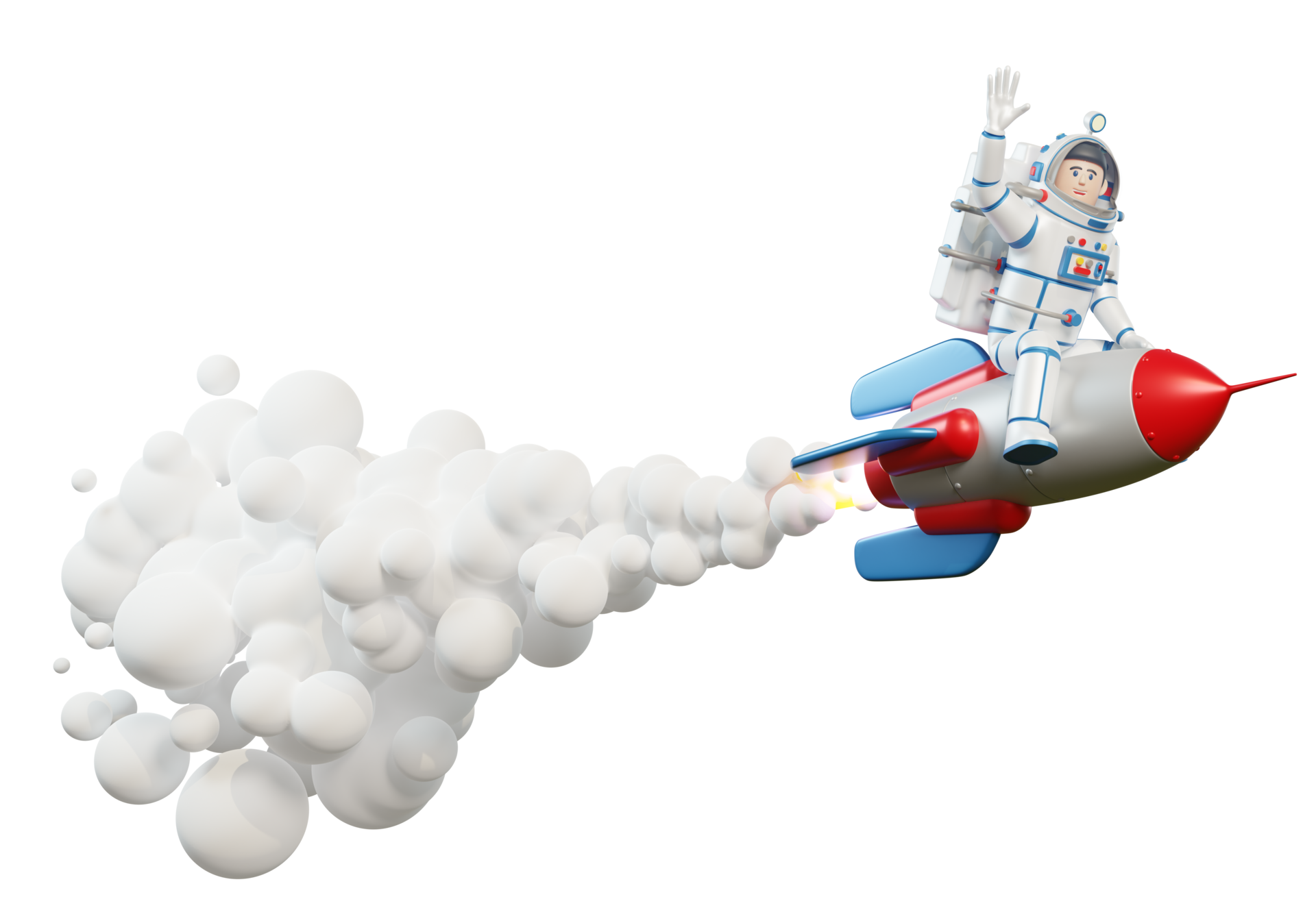The image is a detailed, cartoon-style 3D rendering of a rocket ship with a man in an astronaut uniform sitting on top. The silver cylindrical rocket has a sharp, red-tipped nose cone and vibrant blue wings at the rear. From the rocket's engine, a large cloud of smoke emanates, composed of interconnected white spheres, almost resembling marshmallows, with a yellow glow where the smoke begins. The astronaut, who appears as a small toy figure resembling a Lego, is dressed in an all-white suit with blue striping and a control panel on his chest adorned with yellow, red, and gray knobs. His helmet is open, revealing a cartoonish Caucasian face with black hair. Straddling the rocket as if riding a horse, he waves cheerfully with one hand, inspiring a sense of joy and whimsy.